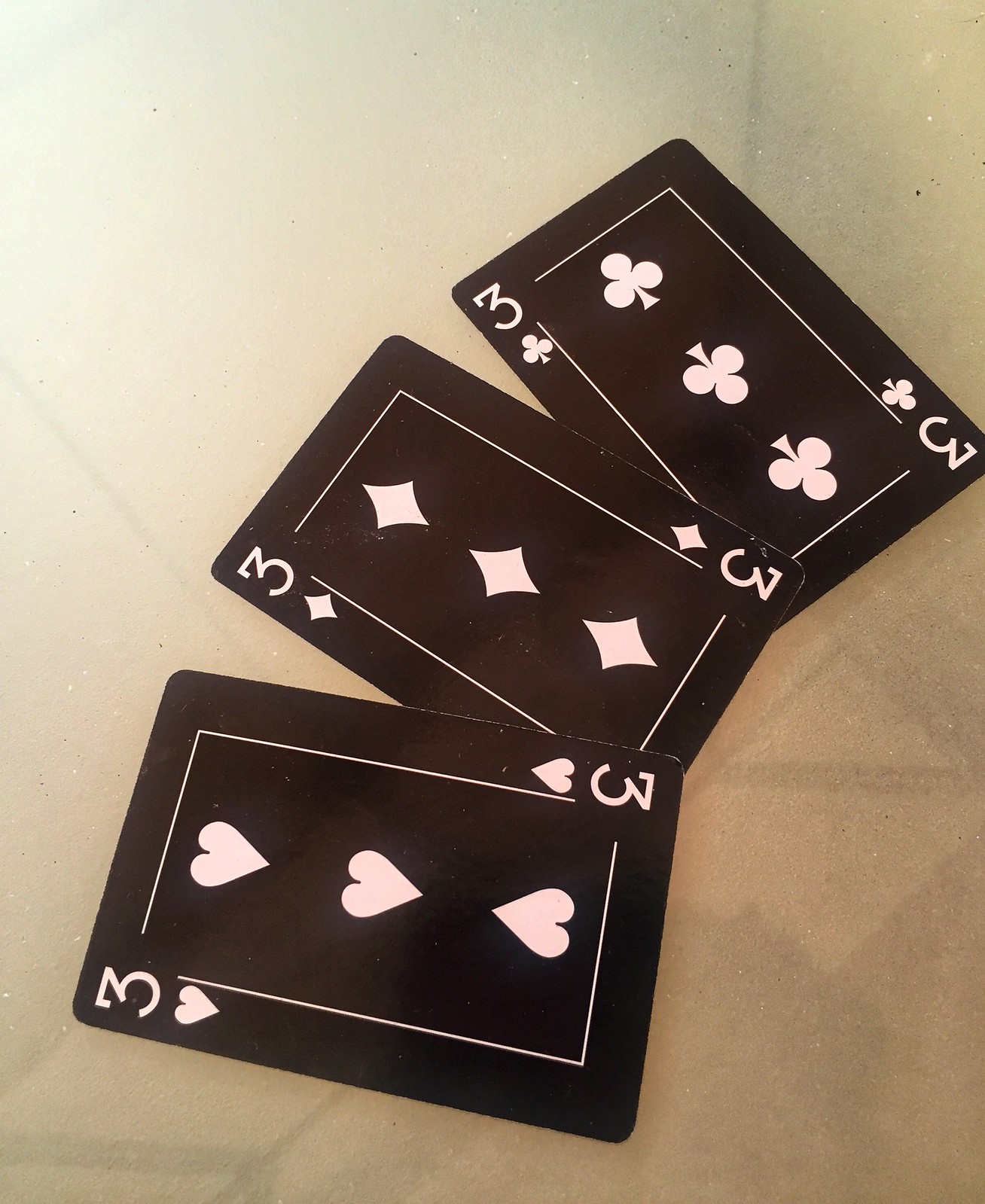The image captures a unique set of playing cards displayed on a surface that appears to be either wood or tile, though the perspective does not clearly determine this. The cards are strikingly distinctive, designed with an entirely black background and contrasting white text. Each card features a non-traditional design with white borders forming two L-shaped lines at the corners, creating incomplete rectangles that leave gaps where numerical values are displayed.

Three cards are prominently shown, all of which are the number three but of different suits. The arrangement starts with the three of hearts at the bottom, slightly askew and nearly horizontal, overlaid on the middle card, which is the three of diamonds positioned at a 45-degree angle. The topmost card is the three of clubs, partially visible and turned between 45 and 90 degrees off center.

The minimal overlap of the cards ensures that each suit symbol—a heart, a diamond, and a club—is clearly visible. The overall orientation of the cards creates a visually dynamic spread, emphasizing their bold, monochromatic design.